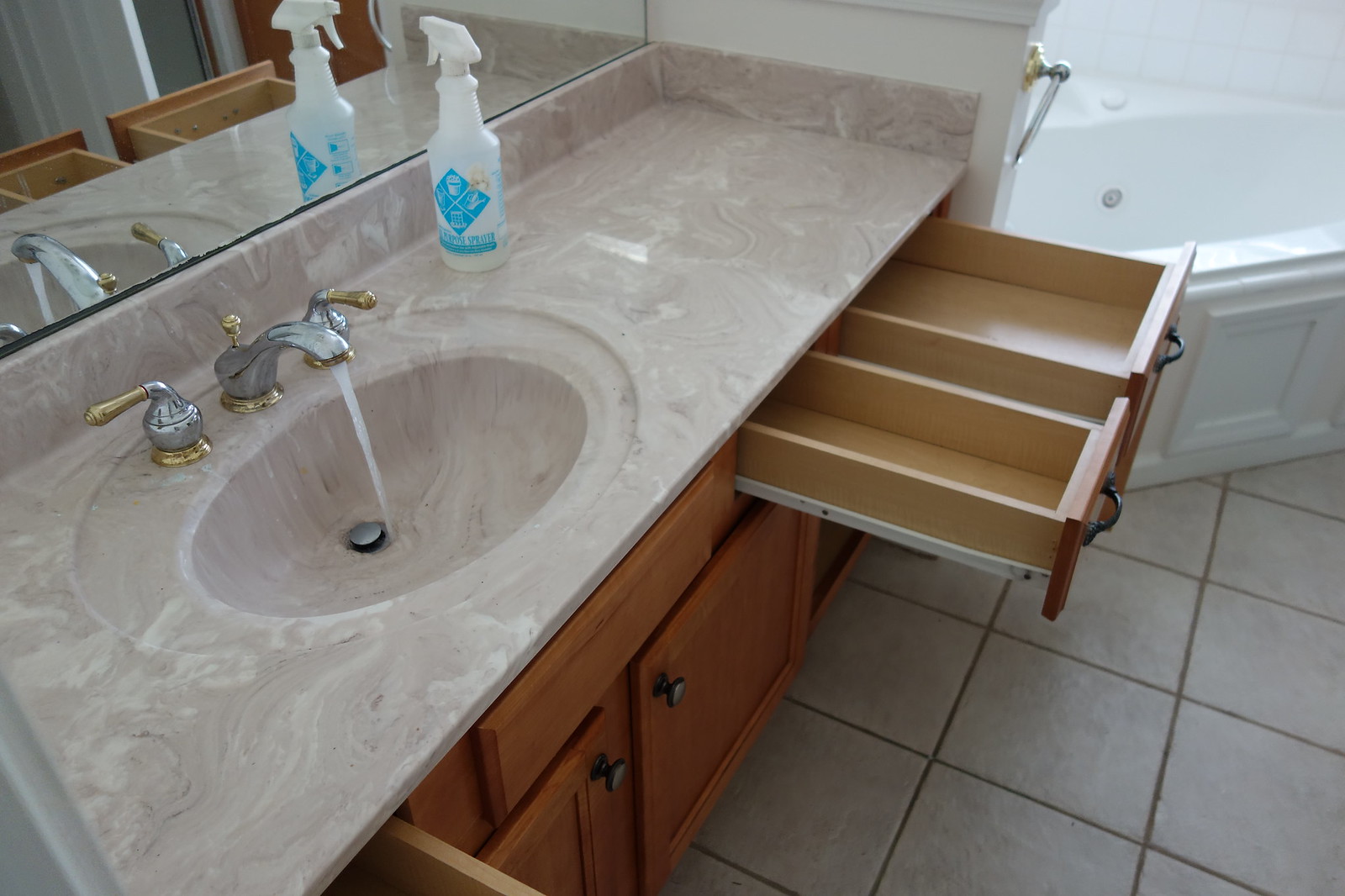The bathroom in the image has a distinctly dated appearance, characterized by several retro design elements. The vanity features tan cabinet doors with a faux drawer located directly beneath the oval sink. Adjacent to the sink are two functional drawers, and there is likely an additional cabinet space beneath those drawers. The countertop exhibits a warm tan hue and is made from a continuous piece of man-made granite, creating a cohesive and durable surface. 

Silver and gold fixtures adorn the sink, adding a touch of vintage charm. Above the sink, there is a mirror mounted on a short backsplash that extends around the back and to the right of the sink area. Interestingly, a blue and white spray bottle is situated on the countertop, suggesting recent cleaning activities.

To the right of the vanity, an octagonal white tub catches the eye, likely illuminated by natural light streaming through a window positioned above it. A silver towel rod with gold-colored bracket fixtures is mounted nearby, adding to the mix of metallic finishes seen in the bathroom.

The front of the tub features a built-in wooden skirt with framed rectangular detailing, blending function with a touch of craftsman style. The flooring consists of oversized tiles with dark grout lines, creating a stark contrast and adding depth to the floor's design. Reflective surfaces and the presence of overhead lighting contribute to a bright and illuminated atmosphere, casting light on the countertop and throughout the room.